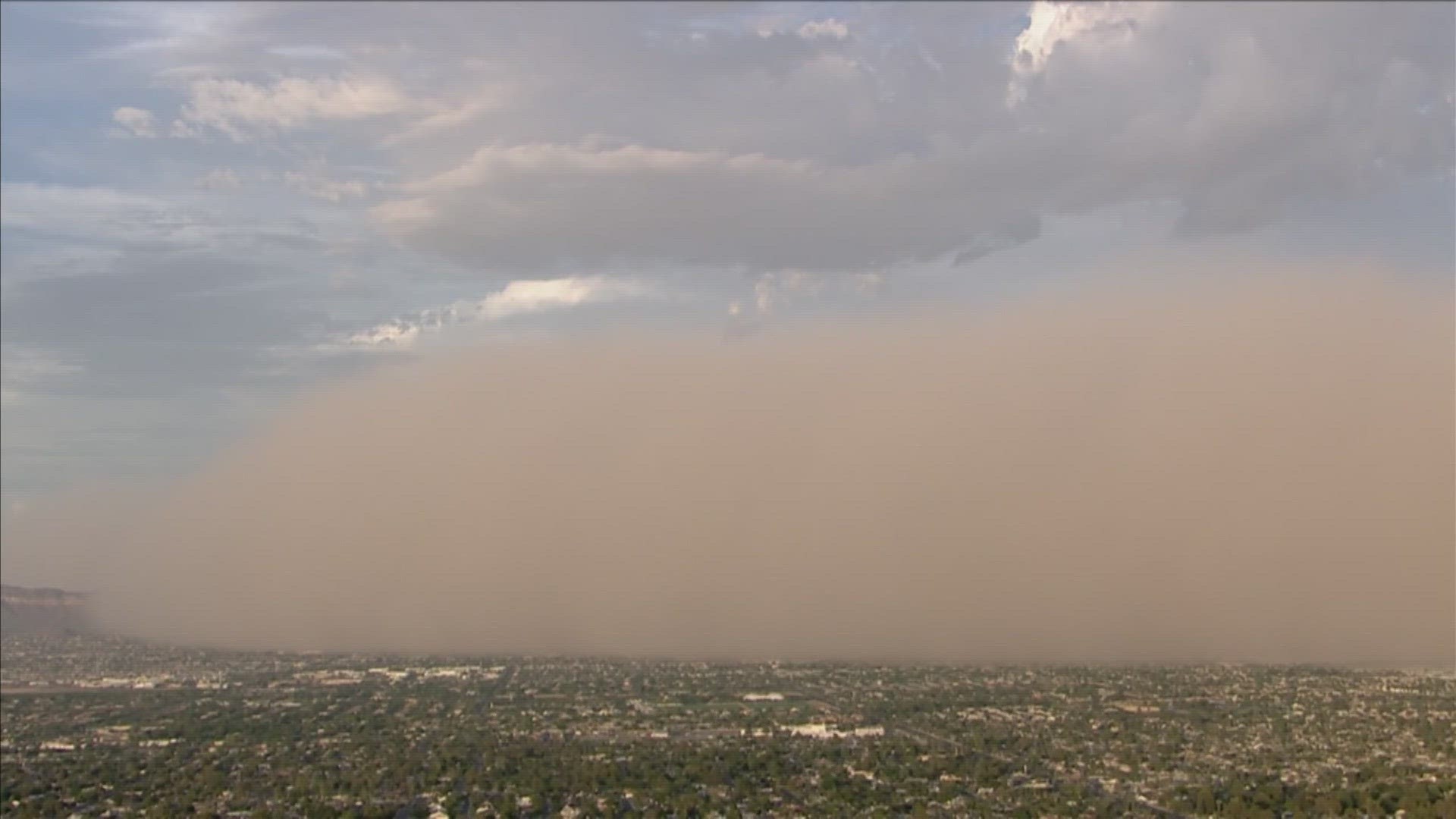This aerial photograph, likely taken during the daytime, showcases a vast expanse of a city landscape from above. The majority of the image is dominated by a blue sky filled with numerous white and gray clouds. Below the sky, the land appears mostly flat and green, interspersed with scattered buildings that populate the city. A significant portion of the cityscape is obscured by a thick cloud of smoke or smog, a light peach or grayish brown in color, creating a distinct haze over the area. The image reveals a stark contrast between the clear sky above and the obscured, hazy city below, framed by numerous trees at ground level.